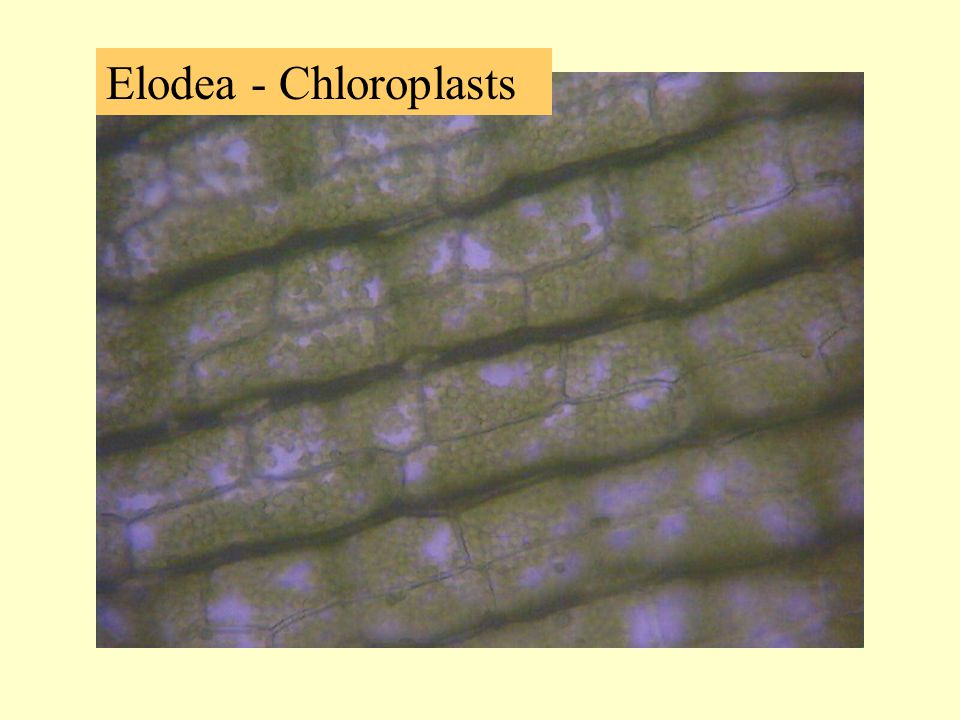The image is framed with a very pale yellow or light brown border and features a dark orange background in the top left corner. Inside the orange box, written in a black serif font, are the words "Elodia Chloroplasts." The main subject of the image is a microscopic, extreme close-up of Elodia chloroplasts, centered within the pale yellow frame. The chloroplasts appear as parallel, horizontal stripes in dark green and white, resembling layers. The cells are organized horizontally and give a textured appearance, akin to a basketball, with distinct white spots scattered throughout. Each cell has a line running through it, contributing to the intricate pattern displayed.